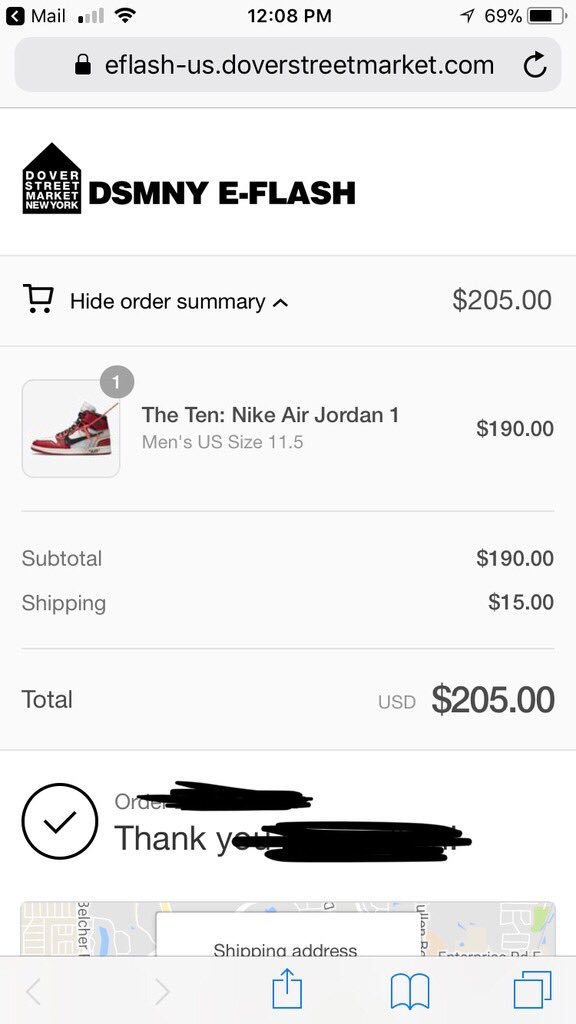**Caption:**

This image is a detailed screenshot of a payment page on a shoe retailer's website, eflash-us.doverstreetmarket.com. The header at the top of the screen displays a white background with various icons: a black box featuring a white arrow pointing to the left labeled "Mail," a single bar of cell phone service, a full Wi-Fi signal (three bars), the time (12:08 PM), a location icon, and a battery icon showing 69% charge.

Directly below this, there is a search bar containing the website URL eflash-us.doverstreetmarket.com, with a back/undo circular arrow and a lock icon indicating a secure connection. The Dover Street Market logo, which looks like an A-frame house, is followed by the text "Dover Street Market New York" in white letters on a black background. Below that, the label "DSMNY E-Flash" appears in black letters.

Moving down, the "Order Summary" section is headed by a shopping cart icon and shows a total of $205. The item listed is a pair of "Nike Air Jordan 1," in men's US size 11.5, priced at $190, with an image of the shoe in red and white to the left. The breakdown of costs includes a subtotal of $190 and shipping fees of $15, summing up to a total of $205 in USD.

Further down, there is a black circle with a check mark inside it. Below this circle, the word "Order" is scribbled out along with the phrase "Thank you," also scribbled out. At the bottom of the section, the text "Shipping Address" appears, accompanied by a small Google Maps image.